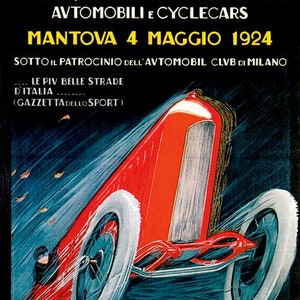The image is a vibrant poster on a black background promoting "Automobile Cycle Cars." The main visual focus is a dynamic scene featuring a red cycle car with distinctive white tires and bluish spokes on its wheels. The front of the car showcases a long, exaggerated grill, and despite its antique design, it resembles modern tractors. The cycle car is depicted in motion, with blue and white speed lines trailing behind and swirling white lines suggesting wind or dirt flying in its wake. There are also small yellow dots scattered to the left of the car, which add a whimsical element to the background.

At the bottom left of the image, there is a small figure driving the car, characterized by black hair, a white face, and sporting a form-fitting black hat, goggles, and a black jacket, suggesting apparel from a period without windshields. The poster includes several lines of text: at the top, "Automobilia Cycle Cars" is written in white font, followed by "Mantova Formaggio 1924" in larger yellow letters. Further down, smaller white text reads "Soto something Parchesino Automobile Civil Milano," with additional unreadable lines below. The overall design evokes a sense of historical racing excitement and technological nostalgia.